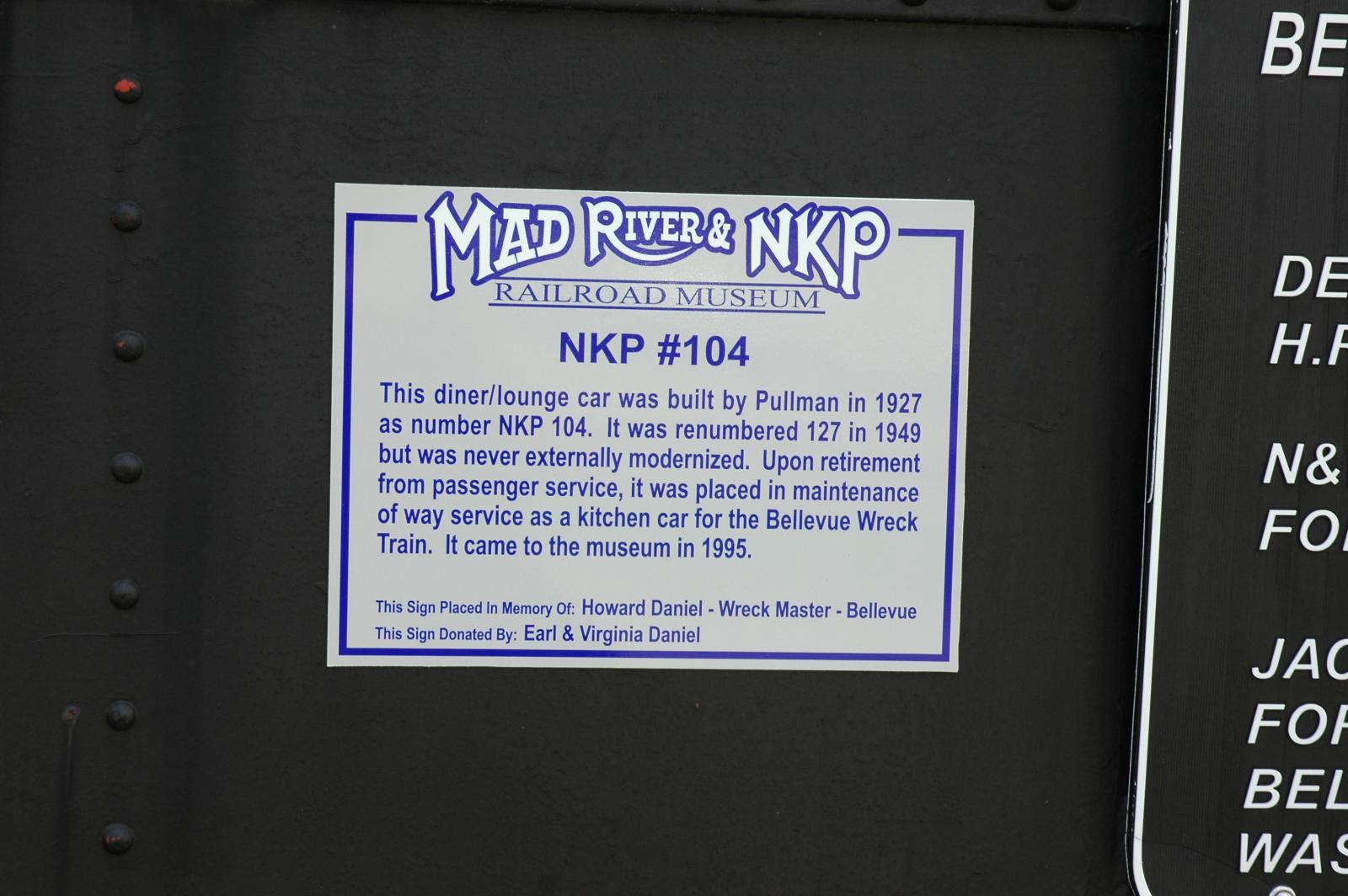The image is a detailed photograph of an informational plaque displayed in a museum. The plaque is mounted on a black painted steel wall, secured with dark tan or gray rivets running vertically along the left side. The plaque features a light gray background with a blue border and blue lettering. The bold title at the top reads "Mad River and NKP Railroad Museum, NKP number 104." Below that, a paragraph provides an overview of a diner lounge car built by Pullman in 1927, initially numbered NKP 104. The car was renumbered to 127 in 1949 but was never externally modernized. After its retirement from passenger service, it was repurposed for maintenance of way service as a kitchen car for the Bellevue Rec Train and was eventually added to the museum's collection in 1995. The plaque also mentions that it was placed in memory of Howard Daniel, a wreckmaster from Bellevue, and donated by Earl and Virginia Daniel. The main colors featured are gray, blue, and white. A nearby black sign with white text is partially visible but cut off.